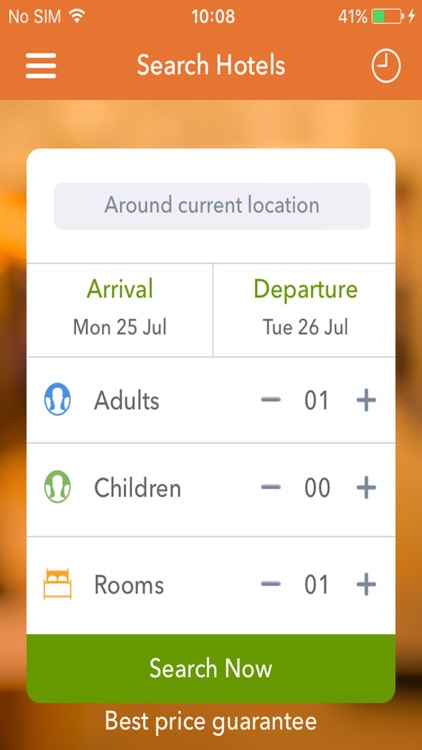This image is a screenshot from a smartphone displaying a hotel booking application. The top border of the screen is orange, and the elements from left to right include:

- A white "No SIM" text on the upper left, indicating there is no SIM card present in the device.
- The Wi-Fi icon next to "No SIM."
- The time displayed in the center as "10:08" without specifying AM or PM.
- A battery icon on the right side, showing a 41% charge with a white lightning bolt symbol, indicating the device is currently charging.

Below this top section, there's another orange strip with "Search Hotels" written in white font. On the left, three white horizontal lines signify a menu option. On the right, a circular icon with a pie-chart-like design represents time.

Further down, there's a white rectangle with rounded corners. At the top of this rectangle, a gray strip features the text "Around current location" in a slightly darker gray font. This section is divided into two columns for selecting dates:

- On the left, "Arrival: Mon, 25 Jul."
- On the right, "Departure: Tue, 26 Jul."

Below this is a gray line with booking details: "Adults: 1," "Children: 0," and "Rooms: 1." Beneath these details, a green rectangle features "Search Now" in white text.

At the very bottom, against the orange background, "Best Price Guarantee" is written in white.